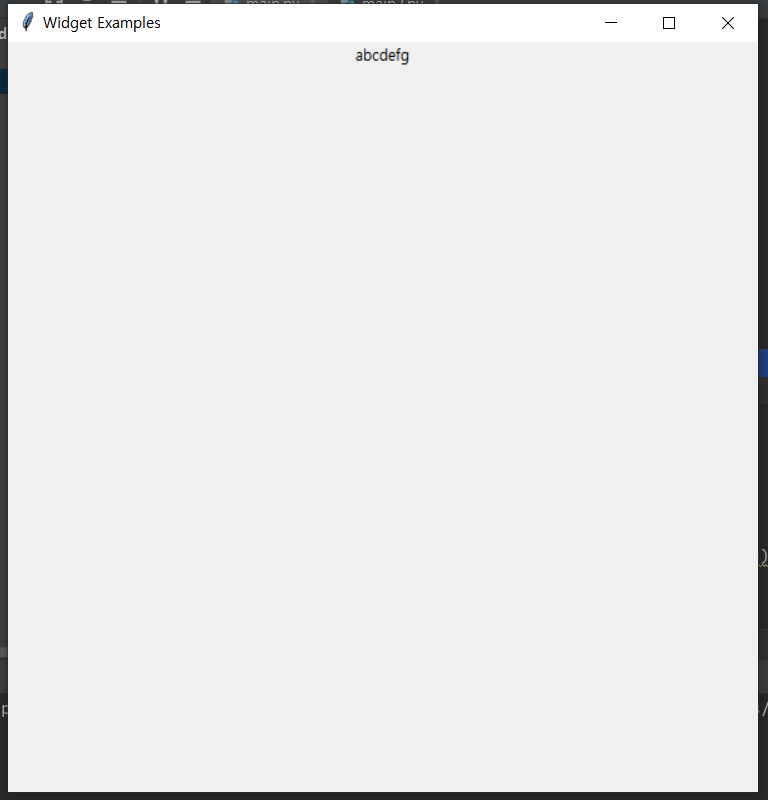Here's a cleaned-up and detailed description:

---

In the image, there is a minimalistic design featuring a very dark black border framing the entire layout. Subtle gray letters that appear to form a "D" and a "P" can be seen, particularly on the left side of the border. 

At the top of the image, there is a white tab. On the left side of this tab is a blue feather icon. To the right of the feather, the words "Widget Examples" are displayed prominently in black text. Further to the right of this text, there is a small box with a square and an X inside it, indicating a close button.

In the center of the image, there is a gray box with black text that reads, "ABCD EFG." This text appears twice in the gray box: "ABCD EFG" and "ABCD EFG." The rest of the image is devoid of any additional elements or text, providing a clean and focused layout. 

Special thanks are extended to Matt and his team for their continuous efforts in managing and producing these visuals.

---